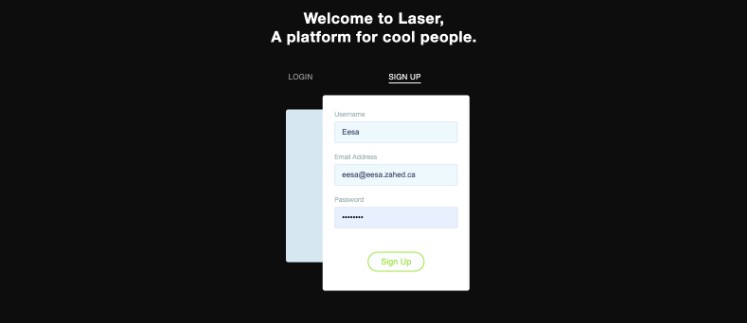A welcome login page for "LazyTown" is presented, specifically designed for a platform that caters to a cool audience. The page includes options to log in or sign up, with instructions to input a username and email address (example: eesa.caegd.ca) and a password, which is denoted by asterisks. To assist users, a helpful link is provided in the description. The sign-up form is housed within a white square, while a blue square, possibly with shades of gray, serves as the background on the left side. This page is characterized as a splash or welcome page for a website, likely indicating a social or community-driven platform. The overall image quality is low, and there is a speculative suggestion that it could either be an actual social website or simply a basic placeholder from someone's initial HTML project.